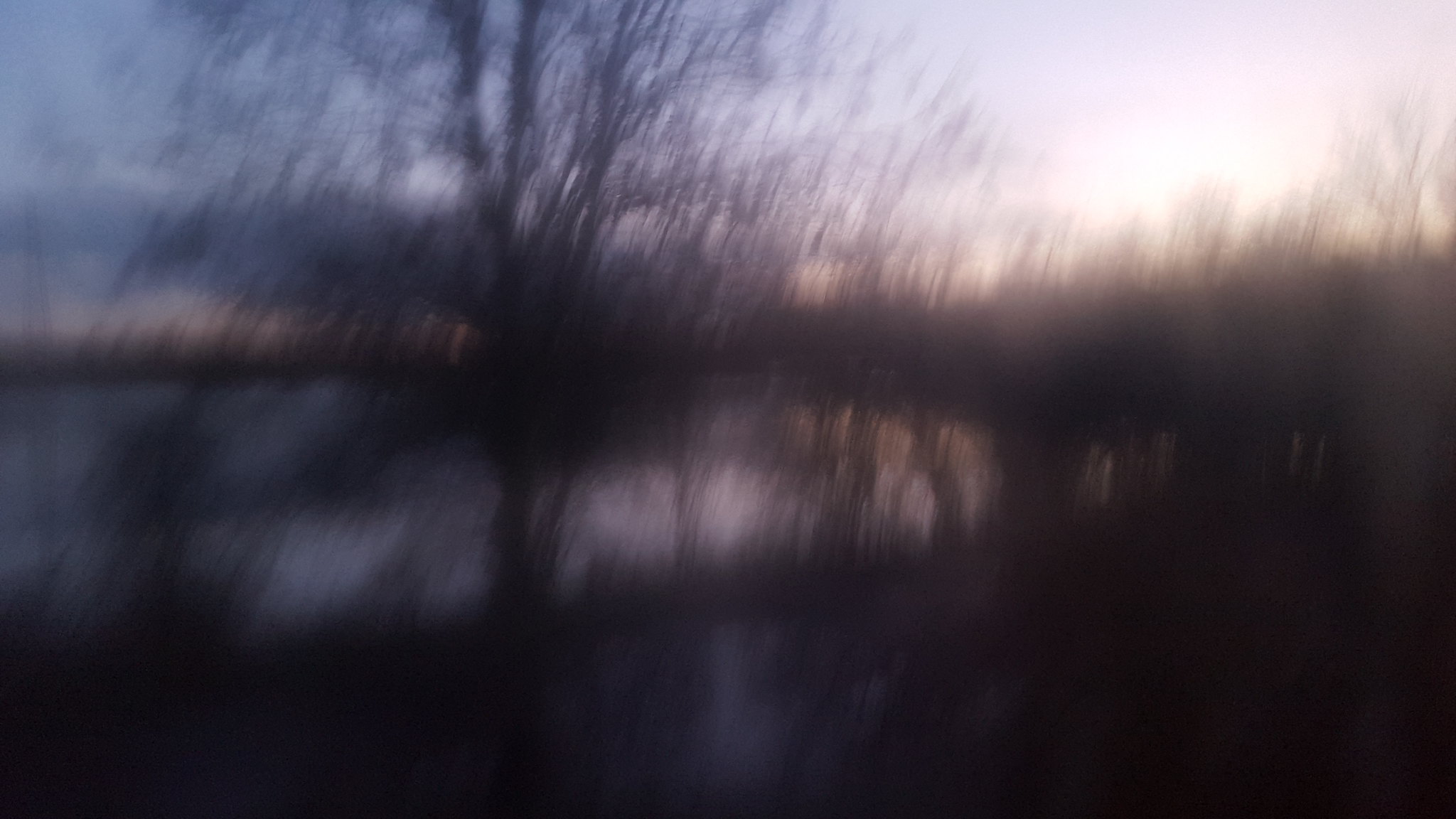This hazy morning photograph, set in the serenity of nature, captures a tranquil scene with a soft, blurred focus. Sunlight peeks over the edge of the leafless, brown-branched trees, casting a bright white and yellow glow that contrasts beautifully against the pale blue sky. The upper left corner of the image features a darker blue hue, adding depth to the sky's palette. In the foreground, a stretch of gray-colored water reflects a sense of calm, offsetting the brown earth tones nearby. Despite the slight blurriness, the image conveys a peaceful and ethereal beauty, evoking the quiet charm of an early morning landscape.